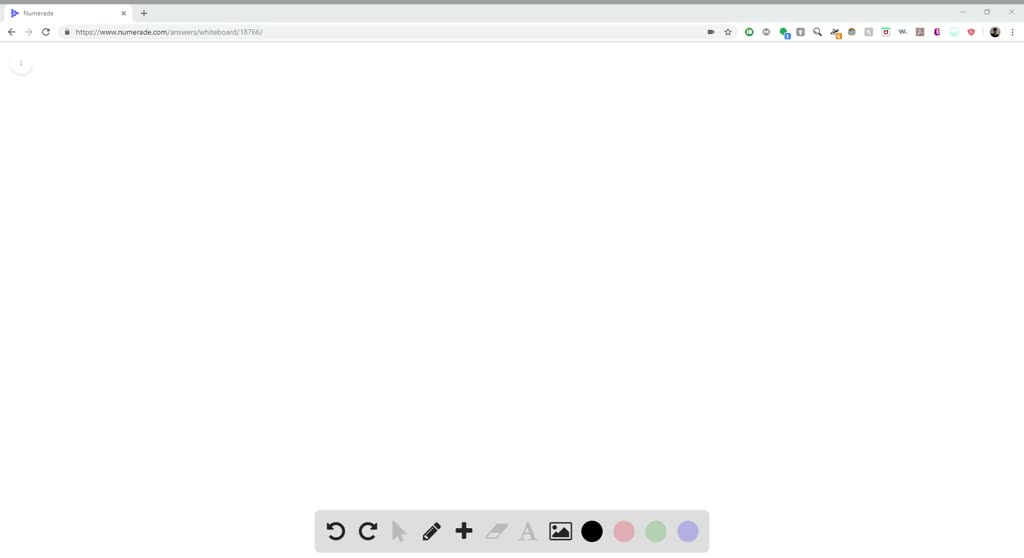In this image, there is a clean, white background serving as the canvas. At the top of the image, there is a blue box with a blue line directly above it, followed by a light blue box. Inside this light blue box, there's a search bar featuring a small blue right arrow and an X icon at the end. Next to it, there’s a left arrow and a refresh (turnaround) arrow. There is another search box located beneath these elements.

Further into the image, we see an arrangement of various small icons. Among them is a circle that contains a person’s picture, accompanied by three vertical dots (indicating additional options). Below this section, a light blue line spans horizontally.

The center of the image is occupied by a large white space. Below this area, there’s another blue box. Within this box, we find navigation arrows including a backward arrow and a forward arrow. Additionally, there’s an upward-left arrow, a pencil icon, a plus (+) symbol, and a small square icon. This section also includes an 'A' letter icon and a black square that depicts an image of a mountain with a sun.

Finally, the image features a set of colored circles lined up horizontally: one black, one red, one green, and one blue.